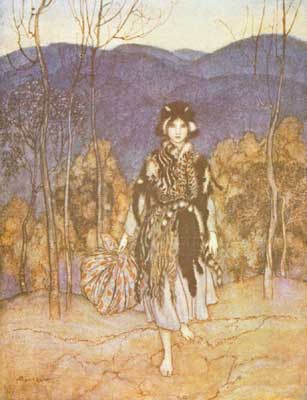This image depicts a detailed painting of a young woman standing barefoot on a yellow grassy terrain. She is walking forward with one leg in front of the other, holding a fabric bundle in her right hand, which appears to contain her belongings. The woman is dressed in a long, tattered, animal-print coat that is black and white, and she also wears a dark hat with her hair tucked underneath. A scarf is tied around her waist. The background features a mix of tall, spindly trees with no leaves and smaller trees in muted browns and golds. In the distance, grayish-blue mountains rise under a slightly sunny and blue sky. The ground beneath her feet shows signs of cracking. The painting includes an illegible signature in the bottom left corner but is undated. The overall color palette consists of vintage shades of slate grays, muted browns, and golds.